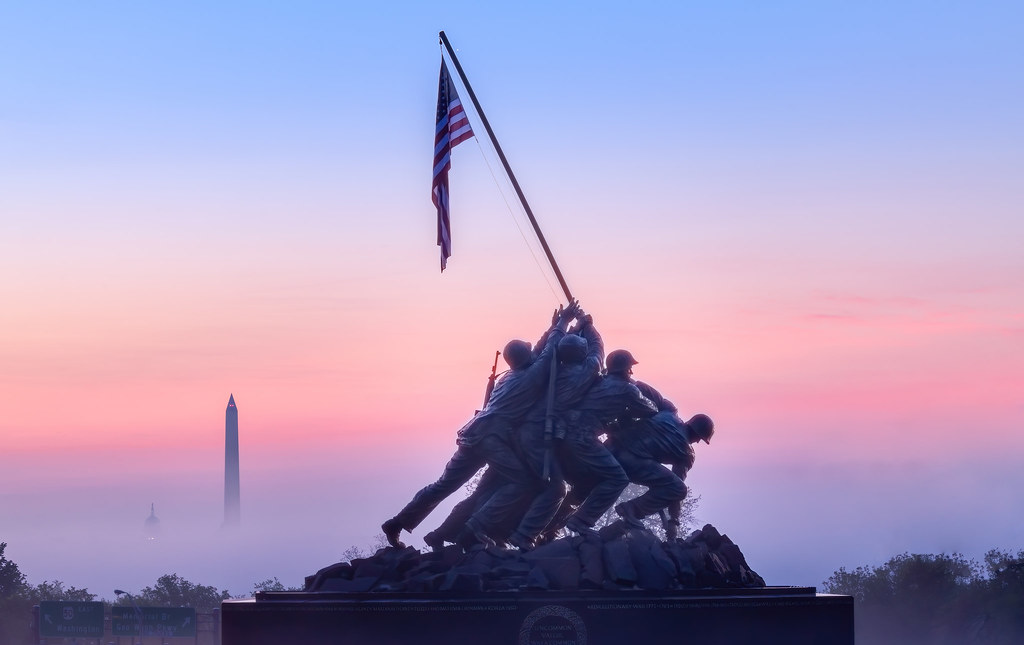This photograph captures the iconic war memorial statue of soldiers raising the American flag at Iwo Jima, located in Washington, D.C. The powerful image shows a group of four to six Marine Corps soldiers, wearing helmets, working together in a pile to plant the flagpole at an angle on what resembles a cliffside. The statue is prominently displayed on a podium and appears to be made of metal, with the flag itself being a fabric American flag hanging down without much wind. The scene is set against a striking sky, transitioning from hazy purple and reddish hues near the horizon to a brighter pink and eventually to a dark blue at the top, suggesting the photo was taken either at sunup or sunset. The background skyline is foggy and hazy, with silhouettes of the Washington Monument and possibly the Capitol Building barely visible through the mist, adding a sense of solemnity and reverence to the memorial.